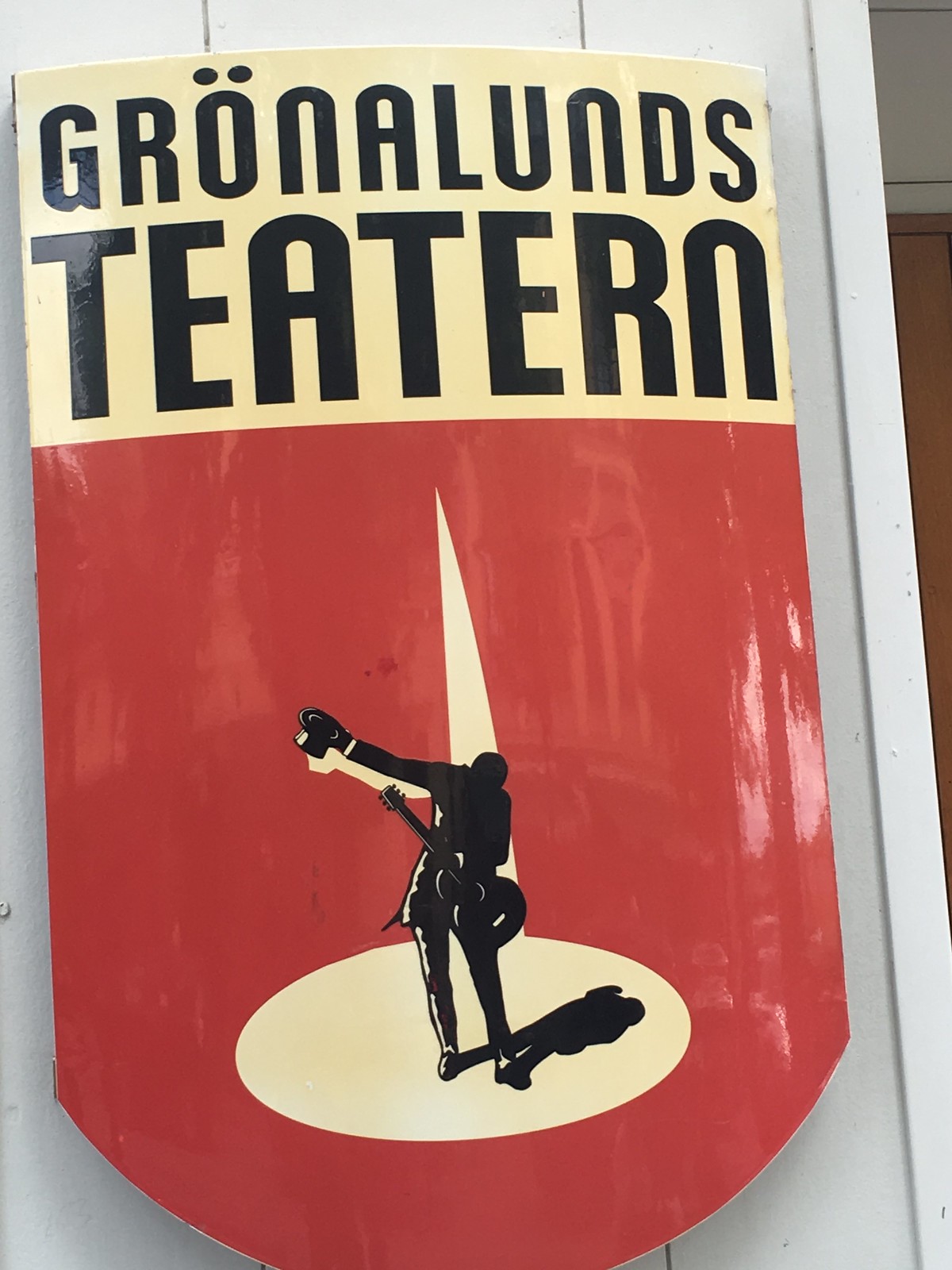The photograph features a promotional sign, beautifully designed in the shape of a shield with straight sides, a slightly rounded top, and an outwardly rounded bottom. The sign, hanging on a white building adorned with a few subtle lines, has a distinctive color scheme: the top third is painted pale yellow while the bottom two-thirds are vivid red. The center of the red section prominently displays the black silhouette of a man bowing, with a top hat extended in his right hand and a guitar nestled under his left arm, all within the shape of a yellow spotlight. Above this striking silhouette, in the yellow section, is the bold, black text 'GRÖNA LUNDS' on the first line, followed by 'TEATERN' on the second line, denoting the sign's association with a theater. This artistic blend of imagery and text strongly signifies a vibrant theatrical or musical venue, possibly situated in a European country.